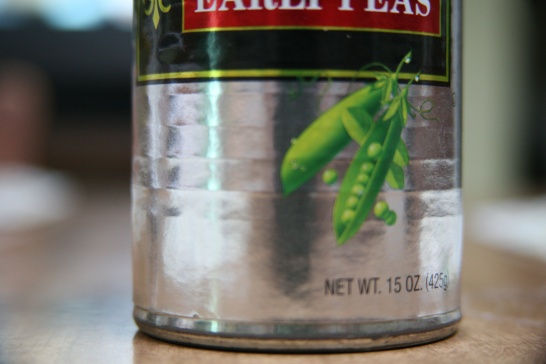This detailed photograph focuses on the lower portion of a 15-ounce can of peas. The can is placed on a tan-colored surface, with noticeable discoloration and browning on its silver bottom. The label on the can features two green pea pods surrounded by individual peas. Above this illustration, the label transitions into a green section trimmed with a gold border, followed by a red section also bordered in gold. While the label's white font is mostly cropped out, the word "peas" remains visible. Additionally, there is a decorative gold icon on one side of the label. Reflections of white light are visible on the can, and the background is partially blurred, depicting an off-white wall.